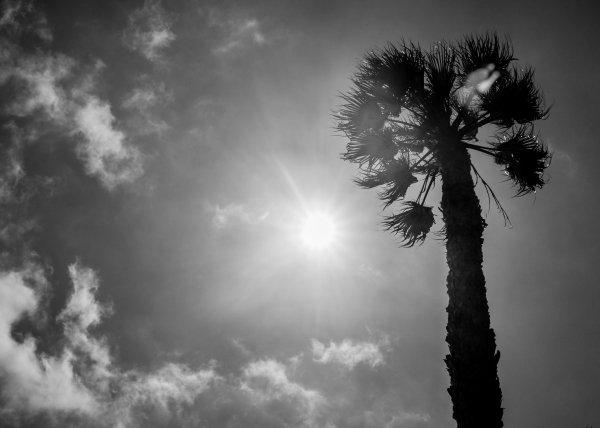The photograph, a black and white image, captures a striking upward perspective from the ground. Central to the composition is the sun, unobscured and glowing brightly in the sky. To the left of the sun, a scattering of small, fragmented clouds creates a sense of mistiness or haze, adding a foreboding tone to the image. Dominating the right side, the tall, slender trunk of a palm tree ascends into view. The tree's many branches extend primarily near its top, each adorned with leaves, suggesting possible movement due to wind. The branches vary in direction, with some reaching upward, others pointing down, and those in the middle extending horizontally. The overall atmosphere is darkened by the image's monochrome filter, lending a dramatic and somewhat eerie feel to the scene.